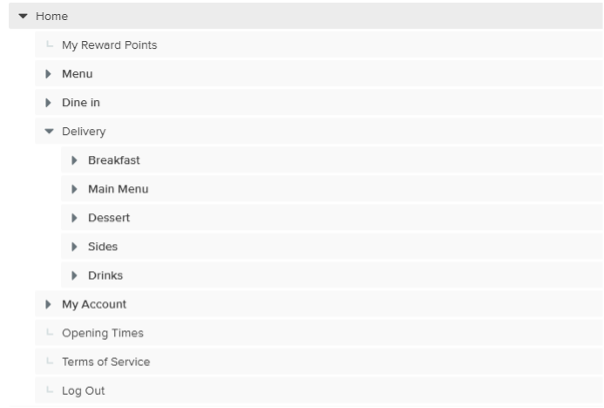The image displays a user interface with a white background and black text. At the top, an icon labeled "Home" has an arrow pointing downward. Below this, you see a menu section, in the following order:

- "My Reward Points"
  
Directly underneath "My Reward Points," there is an arrow pointing to the right leading to a submenu.

- "Menu" (arrow pointing to the right)
    - "Dine In" (arrow pointing downward)
    - "Delivery" (arrow pointing to the right)
    - "Breakfast" (arrow pointing to the right)
    - "Main Menu" (arrow pointing to the right)
    - "Dessert" (arrow pointing to the right)
    - "Sides" (arrow pointing to the right)
    - "Drinks" (arrow pointing to the right)

Following the menu section, there are options for:

- "My Account"
- "Opening Times" (with an open box next to it)
- "Terms of Service" (with an open box next to it)
- "Log Out" (with an open box next to it)

This detailed caption describes the entire contents of the image, set against a simple white background, and features purely text-based interactions.